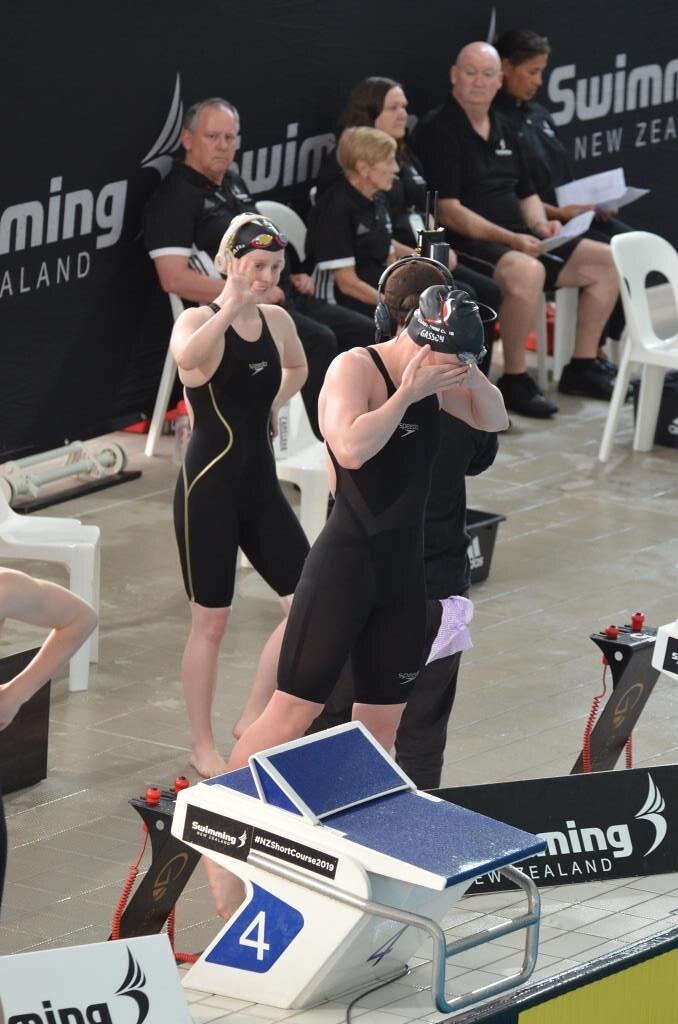The image captures an indoor swimming competition setting. At the forefront, there is a small blue platform with a white base, marked with the number 4 in a blue square. The platform is likely a starting block used by swimmers. A female swimmer is positioned behind it, wearing an all-black, knee-length swimsuit and a black swim cap. Her hands are covering her face, making it impossible to identify her. Beside her, another swimmer, dressed in similar swimming attire and also wearing a cap, is waving her right arm. In the background, there are individuals sitting on white chairs against a dark blue backdrop that repeatedly displays the words "Swimming New Zealand" and "NZ Short Course 2019." The floor beneath them is gray. The scene suggests that the swimmers are preparing for a race, with coaches and other officials seated nearby.